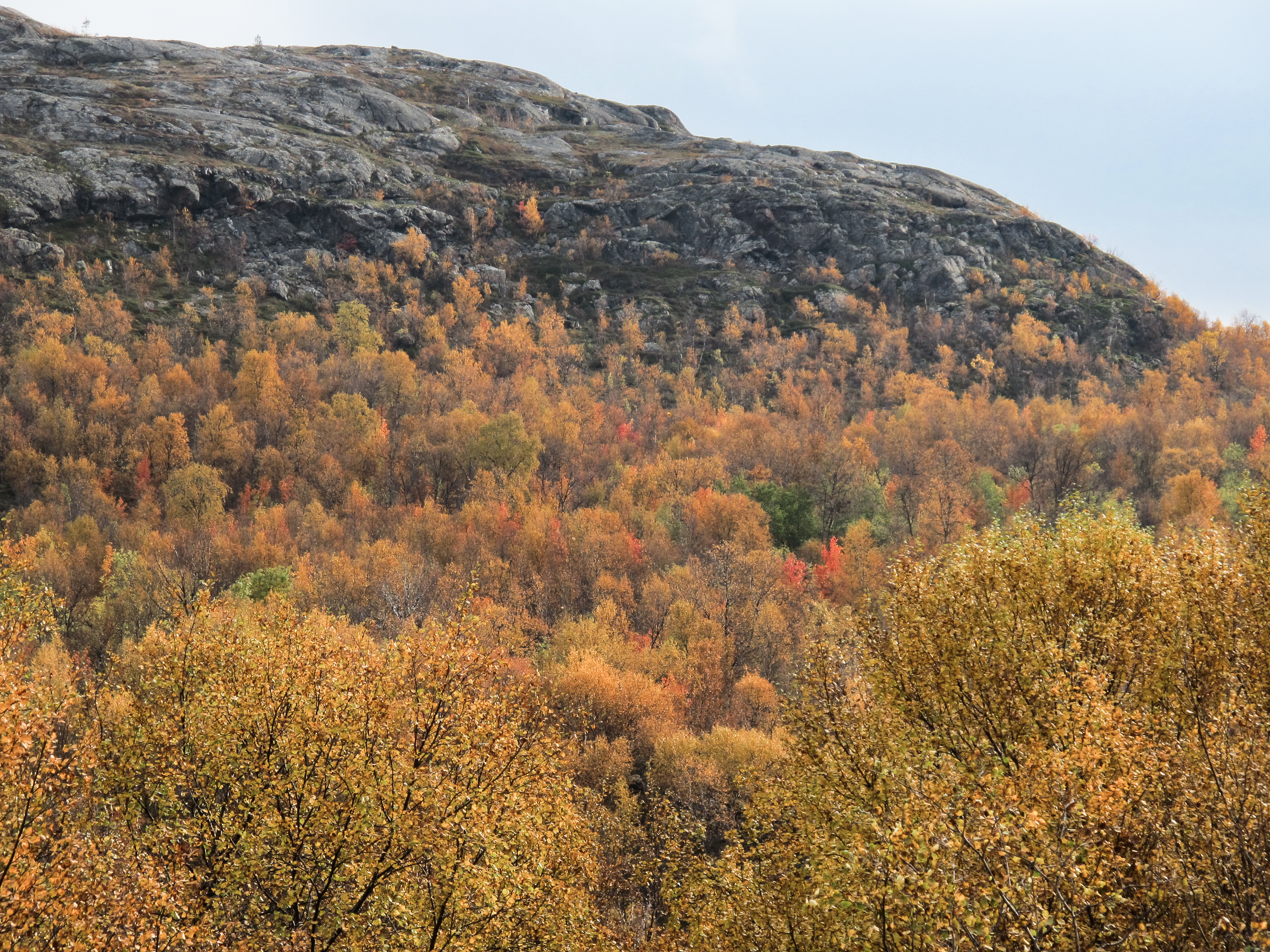The image captures a stunning autumn landscape with a prominent mountain and a dense forest. In the foreground, the trees exhibit a vibrant palette of fall colors, featuring brilliant yellows, reds, and a few lingering greens, suggesting the peak of the autumn season. As the foliage extends halfway up the mountain, the trees become sparse, giving way to a rough, charcoal-gray rocky outcrop that dominates the midground. This rugged mountain is characterized by its bare, solid rock, devoid of significant vegetation except for a few patches of grass. Behind the mountain, a clear, light blue sky, free of clouds, peeks through at the top right corner, adding a serene backdrop to the otherwise dramatic terrain. The image emphasizes the contrast between the vividly colored trees in sharp focus at the front and the rugged, barren mountain that gradually blurs in the distance.